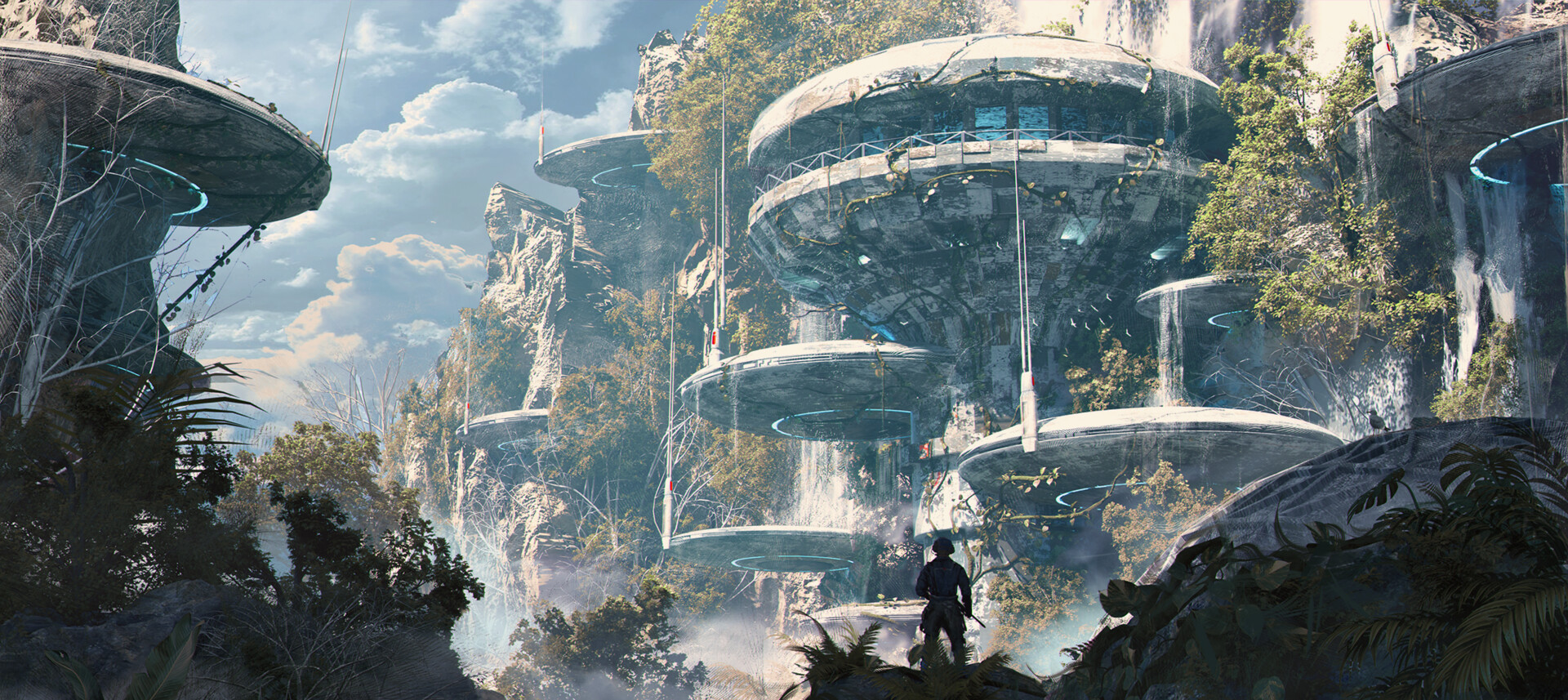A CGI-generated image portrays a futuristic world featuring structures resembling flying saucers jutting out from the side of a barren mountain. These round disk-like houses, about eight in total, are attached precariously to the rocky, gray mountainside and illuminate the scene with blue lights glowing from their undersides. The landscape is dotted with both green scrub growth and dead trees, presenting a stark contrast. On the left side of the image, one of these intriguing structures stands out prominently. In the foreground, a shadowy figure, possibly a soldier wearing a helmet and holding a weapon, adds an element of intrigue and scale to the scene. The overall color palette is washed out, enhancing the image's surreal and otherworldly ambiance.